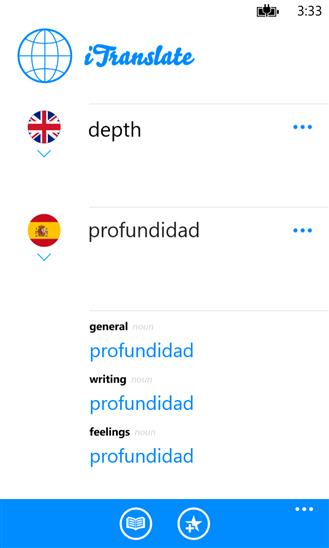The image appears to be a screenshot taken on a mobile phone. At the very top of the screen, the battery icon indicates the phone's current charge level. The time displayed is precisely 3:33. Adjacent to these elements, there is an icon of a globe, designed with intersecting lines reminiscent of a basketball, but colored in blue. The text "i translate" is displayed nearby, with the lowercase "i" and the word "translate" presented in cursive script.

A faint gray line separates this section from the content below. Moving downwards, a British flag is visible next to the word "depth" spelled out as "D-E-P-T-H," followed by three blue, horizontal dots.

Further down the screen, a circular icon shows a red top, red bottom, and a yellow middle, though the exact details within the circle are not clear. Beneath this icon, the word "profundidad" appears, accompanied by the same three horizontal blue dots.

Continuing downward, a list includes the word "profundidad" repeated next to different categories:
- "general, profundidad"
- "writing, profundidad"
- "feelings, profundidad"

At the bottom of the screenshot, there is a blue rectangle featuring a star and a book icon, concluding the various visual elements present on the screen.